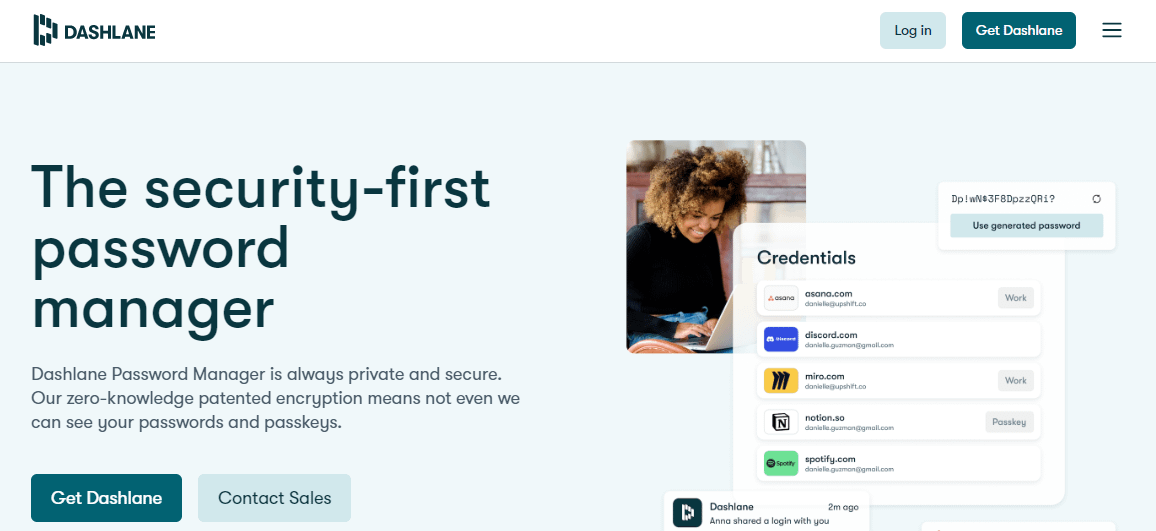This is a left-to-right horizontal image from a website accessible via computer or smart device. The backdrop features a gradient transitioning from white at the top to a pale blue towards the bottom. 

At the top, within the white section, there is a small icon resembling a stylized "D", followed by the text "DASHLANE" in uppercase bold letters. To the right, there are several navigational elements: a "Login" button, a "Get Dashlane" button highlighted in bold teal, and an icon featuring three horizontal lines indicating more options.

Below this, the background shifts to a light blue color. On the left side, prominently displayed in bold text, it reads "The Security-First Password Manager." Beneath this headline, a subtitle explains, "Dashlane Password Manager is always private and secure. Our zero-knowledge, patented encryption means not even we can see your passwords and passkeys."

Further down, there are two clickable options: "Get Dashlane" and "Contact Sales." Adjacent to these options, there is an image of an African-American woman typing on a laptop, accompanied by the text "Credentials."

The credentials section allows users to click on various service entries, including: 
- **Asana.com** (work option available)
- **Discord.com** (no additional options)
- **Miro.com** (work option available)
- **Notion.so** (passkey option available)
- **Spotify.com**

Additionally, there is a note indicating that "Anna shared a login with you two months ago."

Overall, the layout emphasizes ease of navigation and the robust security features of the Dashlane Password Manager.